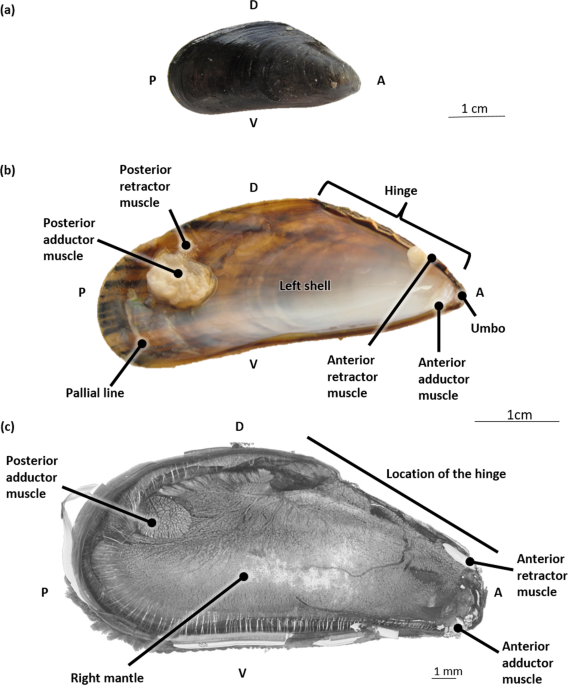The image depicts a detailed anatomical diagram of an oyster, divided into three labeled sections: A, B, and C. 

In section A, the diagram presents a closed oyster with a black shell, identifying four distinct regions: D at the top, P on the left, V at the bottom, and A on the right. 

Section B showcases the interior of the left shell of the oyster, emphasizing its brown color with black stripes and detailing the posterior retractor muscle and the hinge.

Section C provides a gray and white X-ray-like drawing of the oyster, highlighting various internal parts with labels and arrows, including the posterior adductor muscle, posterior retractor muscle, hinge, anterior retractor muscle, anterior adductor muscle, ombo, and the right mantle. 

Collectively, these sections offer a comprehensive view of both the external and internal structures of the oyster.